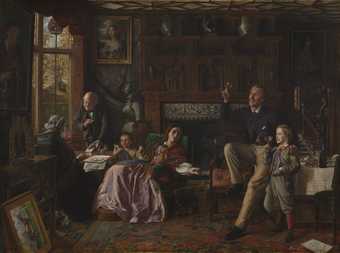This image features a detailed, dark, and moody oil painting depicting a domestic scene set in the 19th century. The central focus is a room with multiple figures and rich interior details. On the left side, an older bald gentleman stands near a window, beside a seated older woman with gray, curled hair in a kerchief. They face a large table that separates them from the other figures. To the right of the woman, a young girl in a long dress sits attentively in a green chair. Further to the right, a man dressed in a dark suit jacket and tan Regency-style pants sits with his leg propped up on a chair, examining an object in his hands. Beside him, a little boy, perhaps in a Boy Scout-style outfit, eagerly looks at the same object. The room itself is decorated with numerous portraits, cabinets, and possibly even a suit of armor, suggesting a wealthy and historic ambiance.